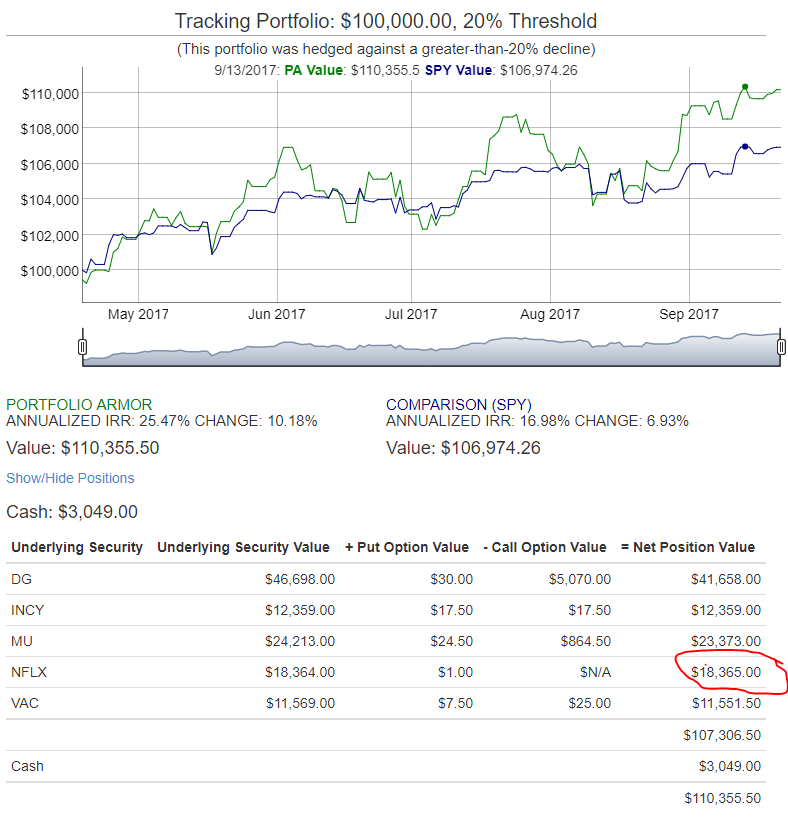The image displays a detailed overview of a tracked portfolio along with comparisons and specific financial metrics as of September 13, 2017. The background is predominantly white, featuring predominately text and a couple of graphs. Here is a detailed caption for the image:

---

**Portfolio Overview as of September 13, 2017:**

- **Header:** The title at the top reads "Tracking Portfolio, $100,000, 20% threshold,” indicating that the portfolio is monitored with a 20% decline threshold. It is mentioned in brackets that this portfolio was hedged against a greater than 20% decline.

- **Date and Values:** The date "9/13/2017" is displayed with two distinct valuation figures:
  - PA Value: $110,355.50
  - SPY Value: $106,974.24

- **Graphical Representation:** Below the text, there is a line graph with two colored lines—a green one and a blue one. Y-axis values range from $100,000 to $110,000, while the X-axis is labeled from May 2017 to September 2017:
  - Both lines start at $100,000 and trend upwards.
  - The green line ends around $110,000.
  - The blue line ends approximately at $107,000.

- **Additional Graph:** Below the main graph is a smaller graph with no specific numerical annotations. It appears as a grey line and bar chart gradually moving upwards.

- **Portfolio Metrics Table:**
  - **Left Column (Portfolio AMOR):**
    - Annualized IRR: 25.47%
    - Change: 10.18%
    - Value: $110,355.50
  - **Right Column (Comparison SPY):**
    - Annualized IRR: 16.98%
    - Change: 6.93%
    - Value: $106,974.26

  - **Show/Hide Positions Option:**
    - Cash available: $3,049

- **Detailed Financial Breakdown Table:**
  - **Headings:** Underlying Security, Underlying Security Value, Plus Put Option Value, Call Option Value, Equals Net Position Value.
  
  - **Underlying Securities Values:**
    - DGIN: $46,698
    - CYM: $12,359
    - UNFL: $24,213
    - XVAC: $18,364
    - Cash: $11,569

  - **Put Option Values:**
    - $30, $17.50, $24.50, $1, $7.50

  - **Call Option Values:**
    - $5,070, $17.50, $864.50, Not Applicable, $25

  - **Net Position Values:**
    - $41,658, $12,359, $23,373, $18,365, $11,551.50
    - Subtotal: $107,306.50
    - Cash: $3,049
    - Total: $110,355.50

This detailed descriptive caption conveys the essence of the image, conveying key financial information and metrics clearly.